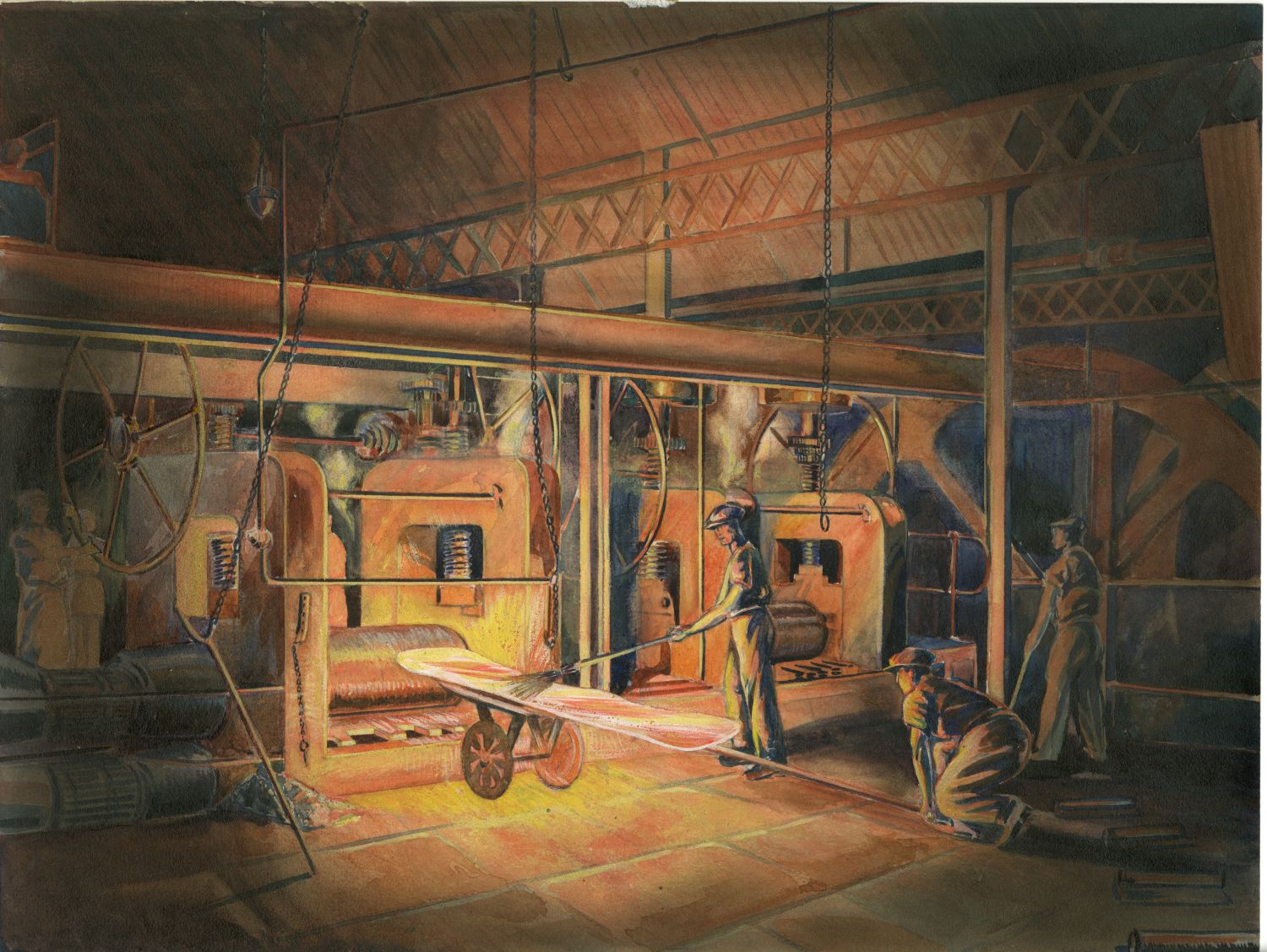The painting is reminiscent of Edward Hopper's style, characterized by light streaming in and creating contrasts in an industrial setting, likely an iron foundry or steel works. The scene is set inside a large, dimly lit factory featuring a slanted roof and heavy machinery, including pulleys and chains hanging from the rafters. The environment is bathed in shades of rosy brick red with illuminating touches of yellow, orange, and white, reflecting the heat and light of ongoing work. Central to the image are three workers clad in informal, 1930s-style baggy clothing and newsboy caps. One man is shoveling material from a cart into what seem to be furnaces, while another, kneeling on the floor, appears to be managing the machinery, possibly a roller and ensuring the process runs smoothly. The third figure on the right is holding a broom, seemingly sweeping debris. The walls exhibit bluish shading, and the men’s clothing carries similar hues, giving depth to the overall industrial ambiance. The painting captures the meticulous toil and vivid atmosphere of early 20th-century industrial labor.